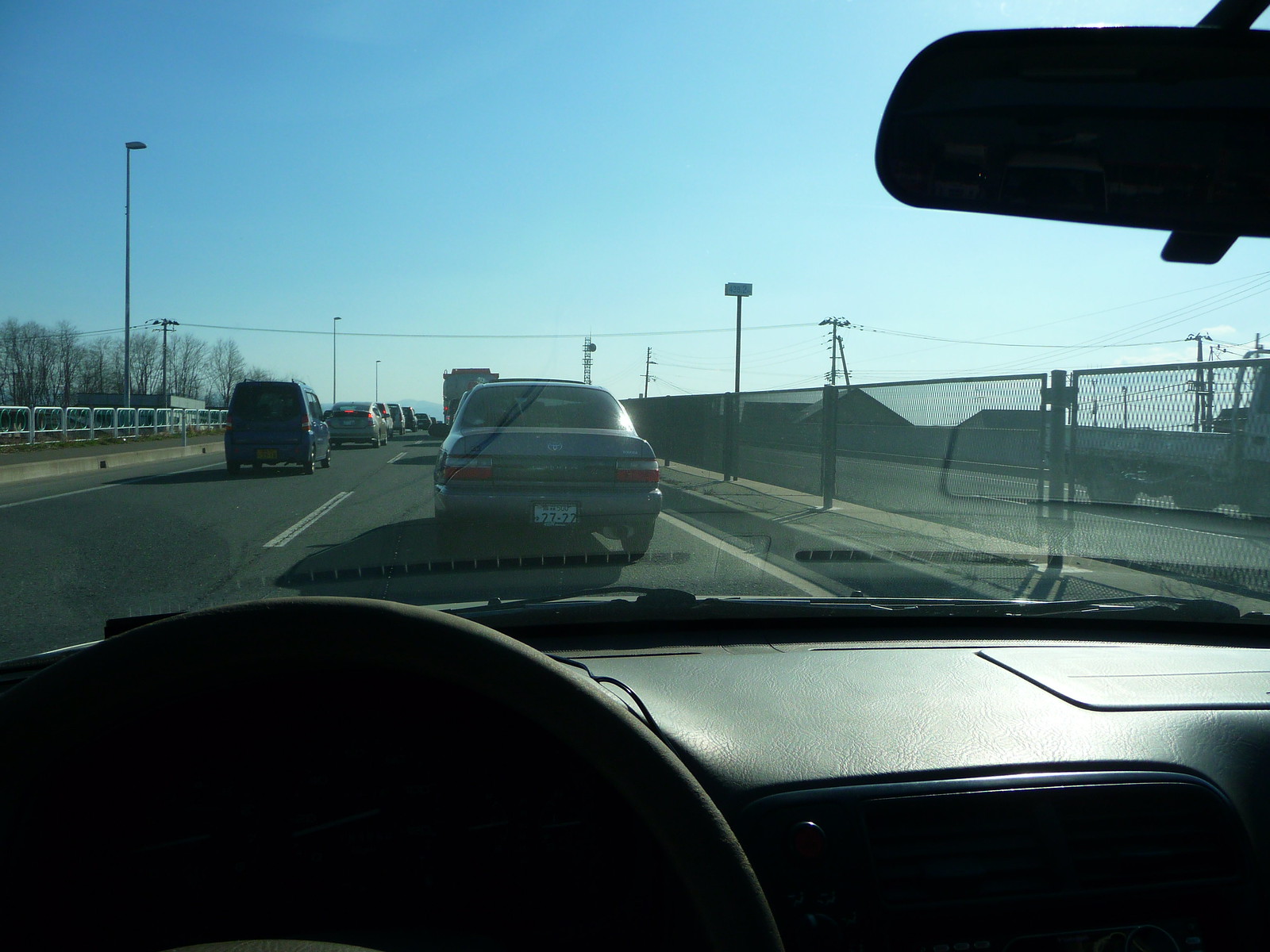The image depicts a vivid scene viewed through the front windshield of a vehicle. Positioned on the left side of the interior frame, the steering wheel and part of the dashboard are visible. The rearview mirror hangs centrally, but due to the dim lighting inside, it reflects nothing discernible. Beyond the glass, it is a bright day characterized by a clear blue sky overhead.

On the road, two lanes of vehicles stretch ahead, both moving in the same direction. The left lane and the right lane are filled with a queue of cars, creating a sense of bustling activity. Flanking the road, different types of fencing are present: on the right side, a rigid wire mesh fence is visible, while the left side is bordered by a more open-plan circular fencing design. 

Tall light poles with lamps mounted on top line the roadway, casting light down onto the vehicles beneath. Additionally, a series of electricity poles run across the entire image, with wires spanning the stretch of the road, hinting at the infrastructure that supports this busy thoroughfare.